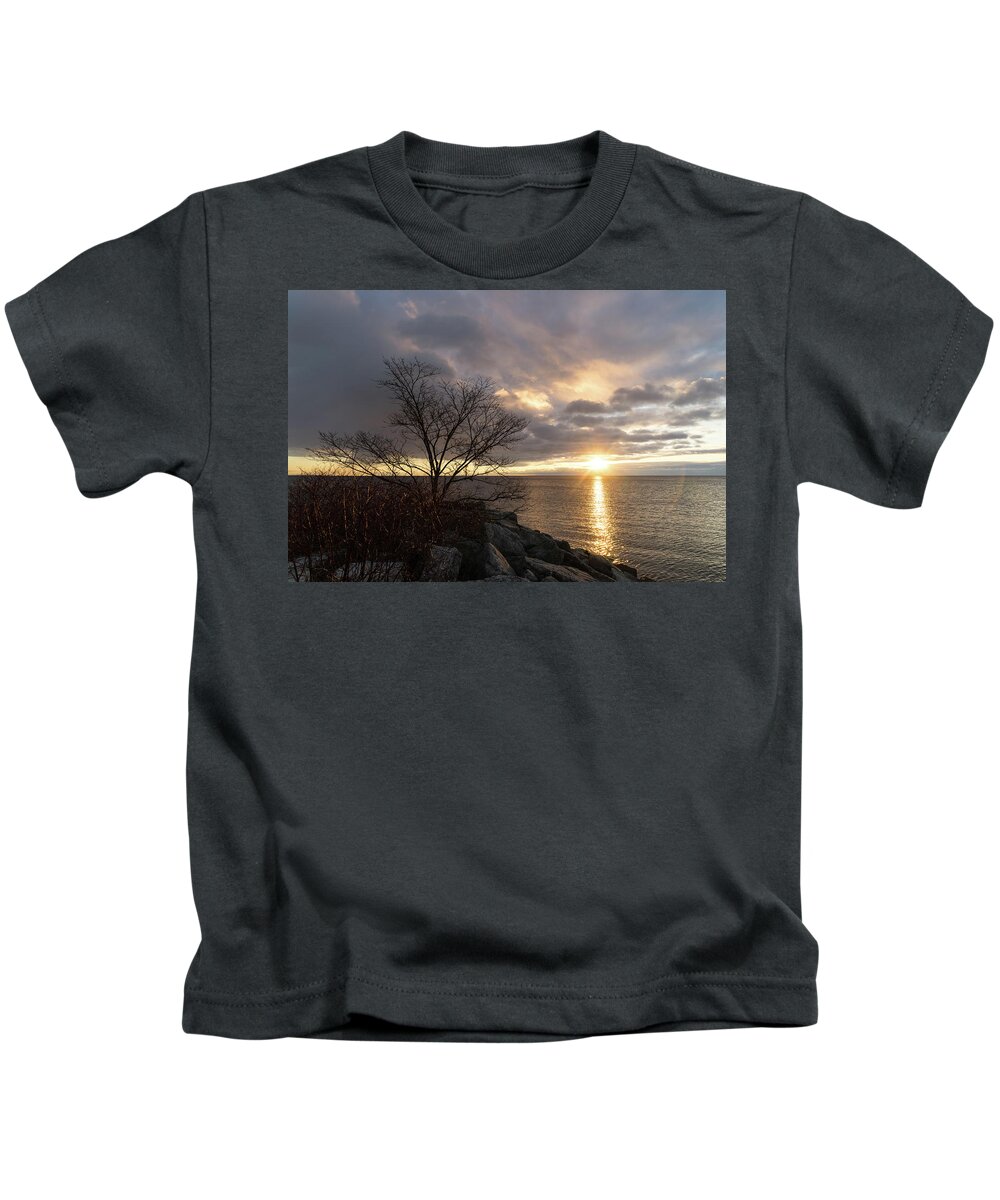The photograph showcases a dark charcoal gray, almost black, short-sleeved crewneck t-shirt. Prominently displayed on the chest is a rectangular image capturing a serene landscape scene at either sunrise or sunset. The sky is filled with purplish-gray and blue clouds, with the sun's orangey-yellow light just peeking from the horizon. This sunlight extends across a calm body of water, casting a muted reflection in the low light. In the foreground, a leafless tree stands on a rocky outcropping, its silhouetted branches reaching upwards. The colors in the image are subdued, primarily featuring grays and blacks for the tree, rocks, and water, creating an evocative and tranquil visual impression.